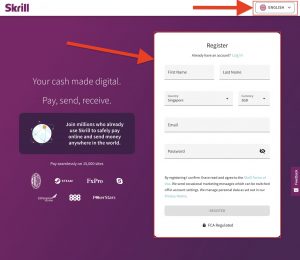The image depicts a screenshot of the Skrill website, primarily featuring a purple-themed interface with white and black text. The word "Skrill" is prominently displayed in a distinctive purple font. A red arrow directs attention towards a drop-down menu that appears to indicate language selection, currently set to "English." Another red arrow highlights the "Register" section, where fields for first name, last name, telephone number, email, and password are visible. The "Register" button itself is currently grayed out, implying it is inactive. 

At the bottom of the form, a lock icon is present, likely signifying security features. Above this section, a slogan in white font reads, "Your Cash Made Digital. Pay, Send, Receive." A black banner spans the top of the purple webpage, adorned with very small white text and a white globe icon. Beneath this banner are several white logos, contributing to the overall sleek and modern design of the website.